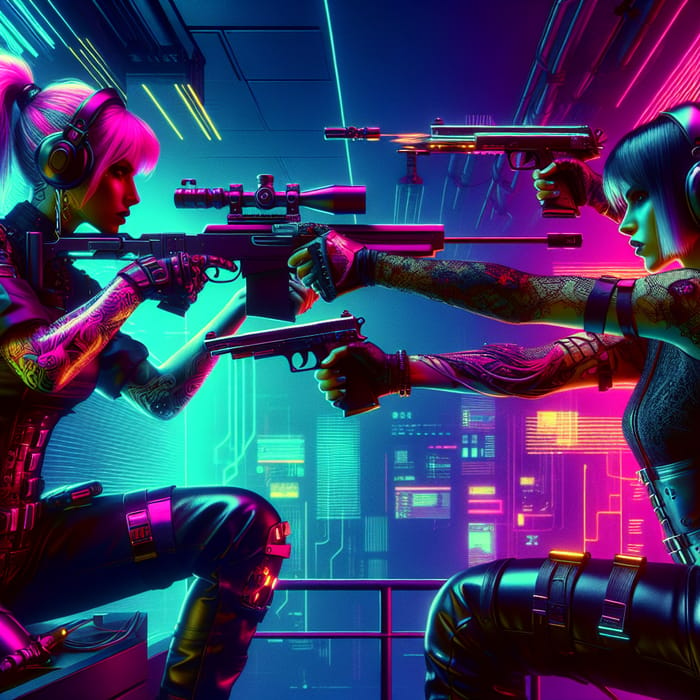In a futuristic fantasy setting, two warrior women face off against each other in a high-tech room filled with machines and lights, reminiscent of a command and control center. The woman on the left, with light blonde and pink hair styled in a ponytail and wearing headphones, is dressed in colorful yet tactical gear dominated by purple and black hues. She sports a fingerless glove on her right hand and grips a scoped rifle with a large clip, aiming it directly at her adversary. The woman on the right, a brunette clad in dark, skin-tight, leather-like armor interspersed with military gear, also wears headphones. Her outfit, predominantly black, is accented by bands around her limbs. She wields a futuristic-looking pistol and revolver, targeting the blonde with calm precision. Adding to the tension, a mysterious third arm holding a .45-style gun emerges from the right side, having just fired a bullet aimed at the blonde woman. The scene is bathed in contrasting colors—pink on the right and blue on the left—emphasizing the standoff's dramatic and perilous nature.